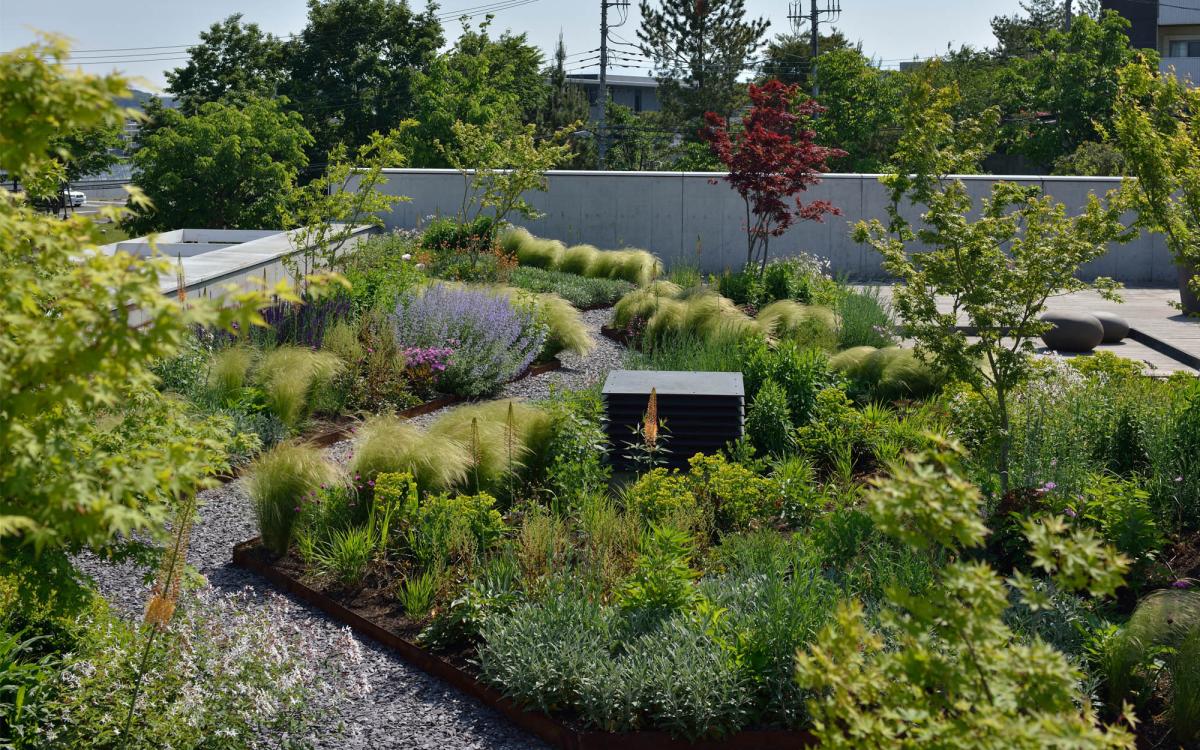The image captures a meticulously landscaped botanical garden, perched atop a rooftop, possibly that of an arboretum or urban building. A winding path of gray gravel meanders through the garden, leading towards a quaint sitting area. This area features large, rounded rock-like structures designed for seating. Dominating the center of the garden is a striking single red tree, standing out amidst a variety of predominantly green plants. To the left of the path, fluffy, light-green bushes contrast with patches of lavender and another purple-hued plant. The garden exhibits drought-tolerant landscaping with varying heights of shrubs and curated foliage, highlighting skilled horticultural planning. In the background, larger trees and telegraph poles rise behind a white barrier, suggesting an urban environment. Other notable details include a black box located centrally and a possible white structure with drawers or slats. The overall scene conveys a serene, well-designed green space, devoid of human presence, meant for visitors to stroll and admire.